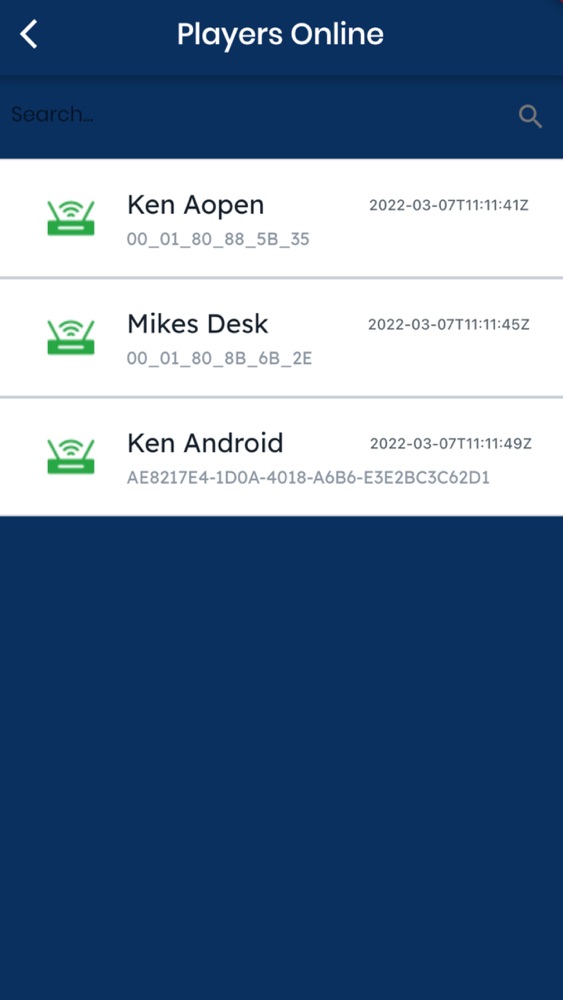Here is a detailed and cleaned-up caption for the image described:

---

The screenshot depicts an online players list interface. The title, "Players Online," is prominently displayed at the top in white font, with the "P" in "Players" and the "O" in "Online" capitalized. The top portion of the interface features a blue background. On the far left, there is a back arrow icon. 

Just below the title, there is a blue search bar. To the left within this bar, the word "Search..." appears in black font, followed by three dots. On the right side of the search bar, there is a magnifying glass icon, indicating the search function.

Below the search bar, the first listed player is "Ken (A-O-P-E-N)," with a number indicating their online status located beneath their name. To the right, the date and time of their last activity are shown. 

The second listed player is "Mike's Desk," with the date and time of their last activity displayed to the right. 

The third listed player is "Ken (A-N-D-R-O-I-D)" with the corresponding date and time of their last activity also noted to the right.